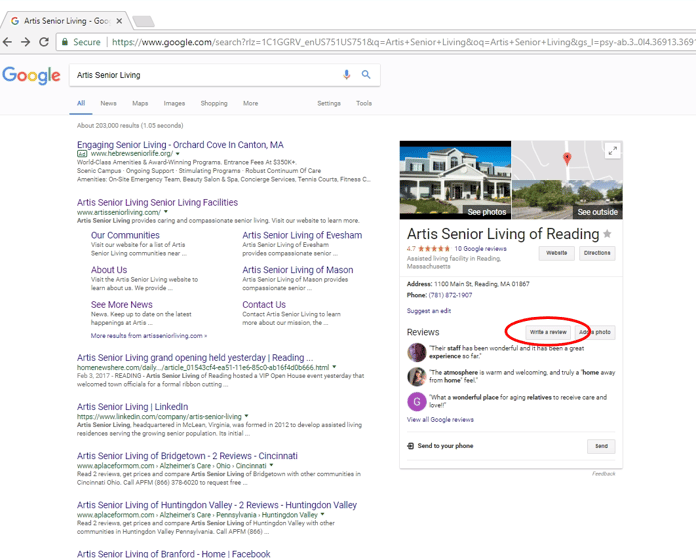**Image Description: Detailed Overview of an Artist Senior Living Search Result**

The image is a screenshot of a Google search result page with a white background, specifically focusing on "Artist Senior Living." The search query results are underlined in blue, signifying clickable links. The top navigation bar contains options such as "News," "Maps," "Images," "Shopping," "More," "Settings," and "Tools."

In the main search results, various details about Artist Senior Living are listed:

1. **Main Headings:**
   - **Engaging Senior Living**: This heading is followed by the location keywords "Orchard Cove" and "Canton, MA."
   - **Artist Senior Living**: This appears multiple times, under different contexts.

2. **Website and Community Links:**
   - **Our Communities**
   - **About Us**
   - **See More News**
   - **Artist Senior Living of Evesham**
   - **Artist Senior Living of Mason**
   - **Contact Us**

3. **Recent News Event:**
   - A notable mention of "Artist Senior Living Grand Opening" that was held yesterday, indicating recent activity.

4. **Additional Locations and Reviews:**
   - **Artist Senior Living of Bridgetown** with associated LinkedIn details.
   - **Artist Senior Living of Reading**, which includes two pictures: one showing the building and another depicting a map with the parking lot.
   - **Artist Senior Living of Huntingdon Valley** with two reviews listed.
   - **Artist Senior Living of Bradford Home**

5. **Social Media and Directions:**
   - Presence on **LinkedIn** and **Facebook**.
   - The Google review section shows an overall rating of 4.7 stars based on 10 reviews.

6. **Interactive Elements:**
   - Two gray rectangles with the options "Website" and "Direction," likely providing direct links to the respective site and navigation details.

This comprehensive search result provides a detailed view of Artist Senior Living's online presence, including multiple locations, recent events, and user ratings, all neatly organized for easy access and further exploration.